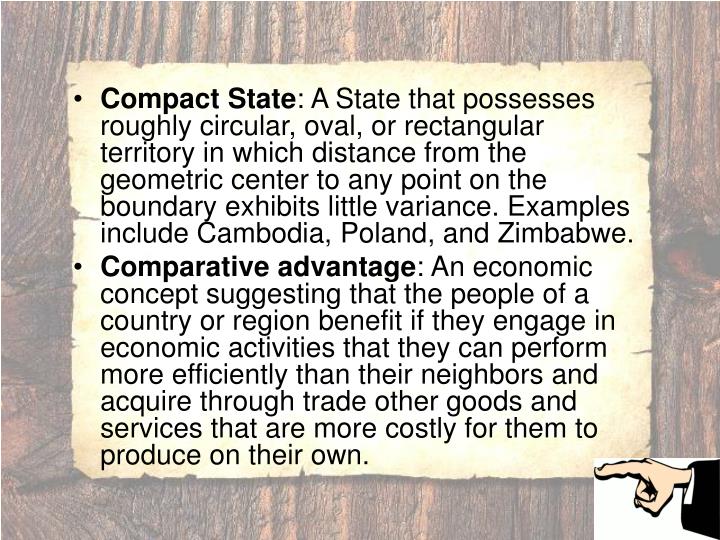The image showcases two detailed bullet points on a white paper background set against a faded wooden table. The first bullet point, labeled "Compact State" in bold, describes a state with a roughly circular, oval, or rectangular territory where the distance from the geometric center to any boundary point shows minimal variance. Examples cited include Cambodia, Poland, and Zimbabwe. The second bullet point, also bolded as "Comparative Advantage," explains an economic principle stating that regions benefit by engaging in activities they perform more efficiently than their neighbors, while trading for goods and services that are more costly to produce locally. In the bottom right corner of the image, a hand, likely that of a white man wearing a black robe, points to the left towards the paper, emphasizing the text.